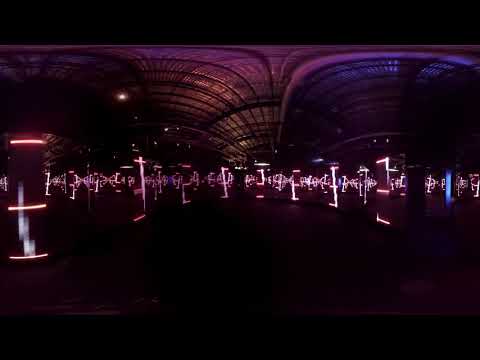The photograph, taken either at night or indoors in low light, showcases an expansive, dark scene dominated by numerous brightly lit objects. The space, which might be an arena, features a patterned ceiling that spans the entire top of the image, with dark lines and a purple hue. The main elements are several standing pillars or posts scattered across the scene, each illuminated with vibrant neon lights, predominantly pink and purple, with occasional blue hues. These light-emitting pillars or statues create a striking contrast against the very dark background, giving the impression of a surreal, otherworldly space filled with glowing figures that extend into the distance. The photograph captures the eerie, mesmerizing glow of these neon-lit pillars, set against the ambiguity of the dark surroundings.